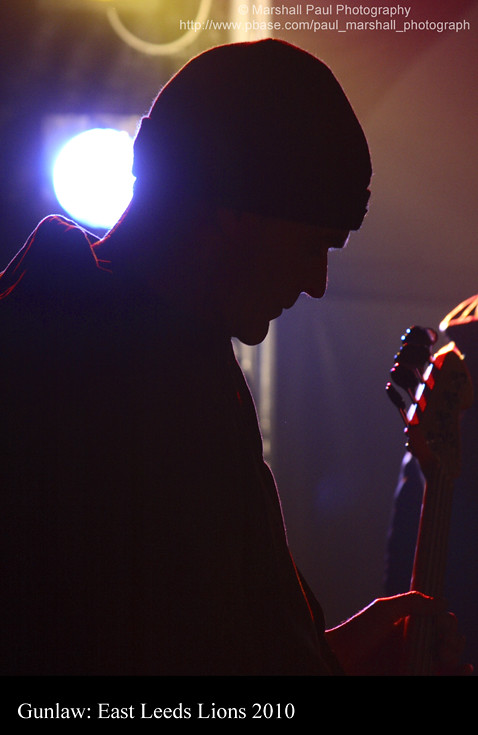In this dark, atmospheric photo, a man dressed in a dark, possibly reddish hoodie and a wool beanie is captured in a profile view, looking downwards. The subdued lighting, pierced by a bright, stage-like spotlight behind him, creates dramatic shadows and highlights, illuminating parts of his face and the neck of his red guitar, which he is holding as he plays. This creates a moody silhouette against the dark background. The setting seems to be a stage or a dimly lit room, with additional blue and yellow lights enhancing the scene. A silver pole is visible in the background, adding texture to the image. At the top of the image, in white letters, it reads "Marshall Paul Photography" along with a website URL. Across the bottom, another text strip in white letters states "Gun Law, East Leeds, Lyons, 2010," contextualizing the event and the performer.